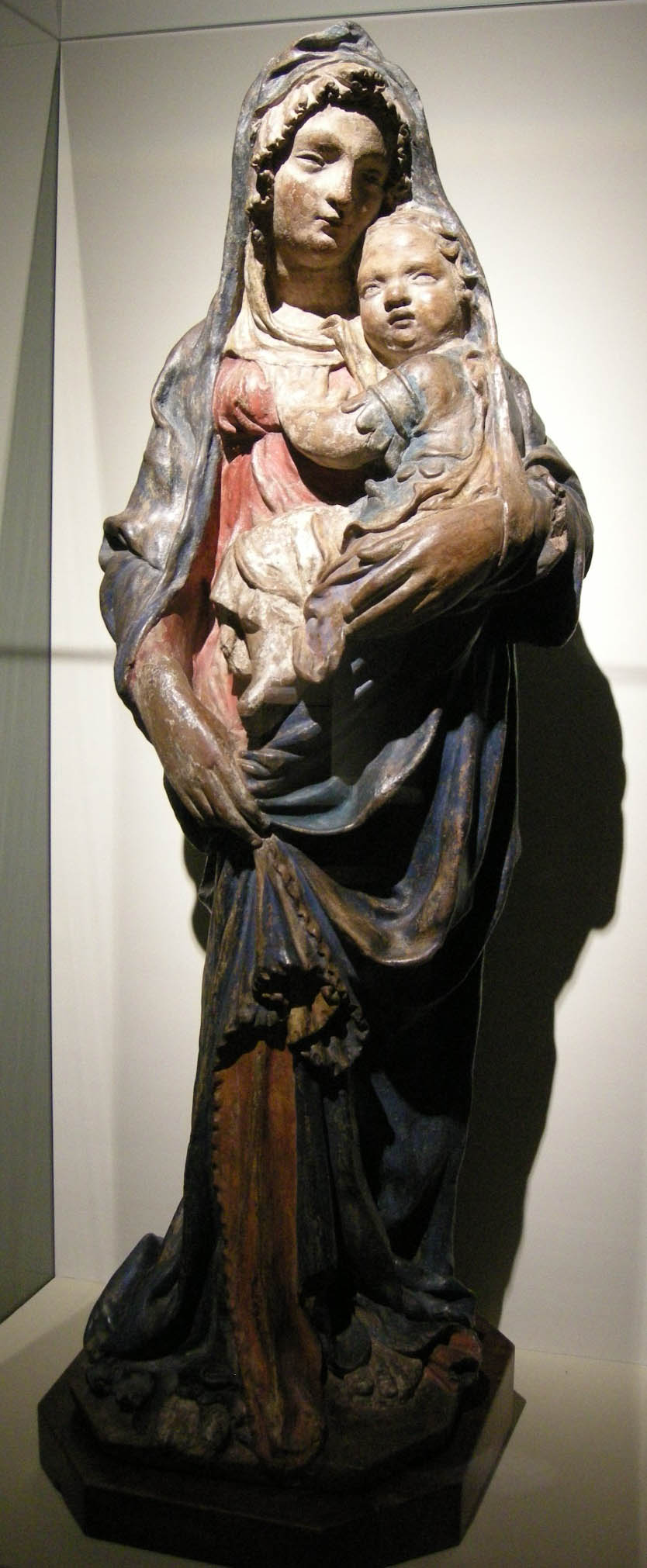This image displays a photograph of a highly detailed statue of the Virgin Mary holding the baby Jesus. The statue, likely made from clay or ceramic and measuring around two feet tall, stands on a square pedestal against a beige-gray background in a museum setting. Mary is depicted wearing a long, blue dress adorned with touches of red, gold, and copper, along with a shawl draped over her head and down past her elbows, rendered in shades of gray and blue. Her face, showing a peaceful expression, is carved with intricate detail, and the same meticulous craftsmanship is evident on the baby Jesus, who also has a calm demeanor. Both have a medium tan complexion. The baby, dressed in blue, is held by Mary's left hand and gazes in the same direction as she does. The statue's drapery work is highly realistic, with loops and folds cascading down to imply a lifelike presence, though Mary's feet are not visible. The overall coloration of brown, blue, red, and copper adds to the statue's aged and serene look.